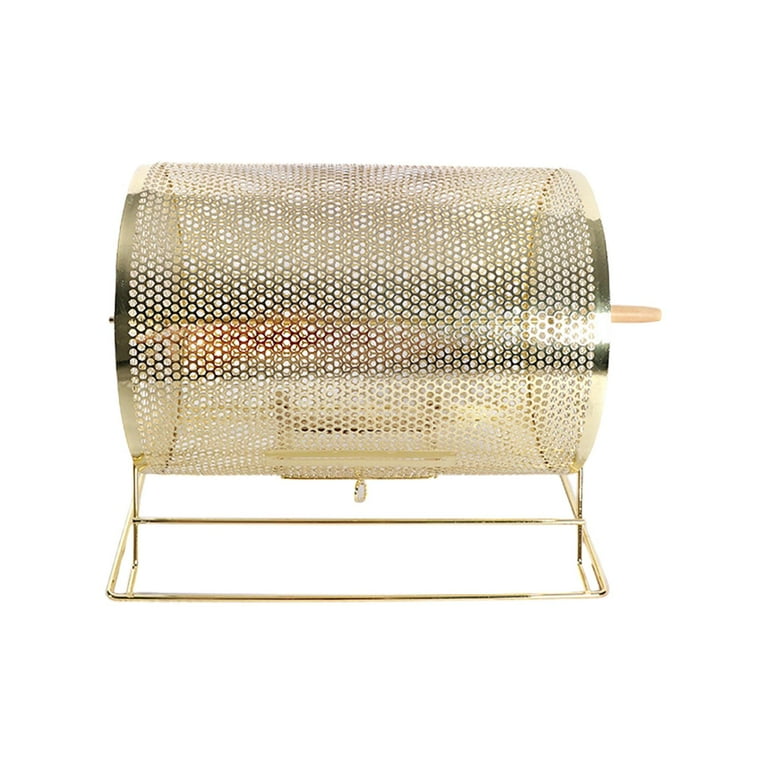The image depicts a gold-colored cylindrical bingo cage, designed for mixing and randomly selecting numbers for bingo or lottery games. The cage is constructed from a mesh-like metal material, making it see-through with numerous small holes on its surface. It stands on a sturdy metal base and features a beige-colored handle on the right side, used to crank and rotate the drum. Additionally, it includes a small trap door at the bottom for retrieving the numbered balls once they have been mixed. The background of the image is plain white, highlighting the object itself.